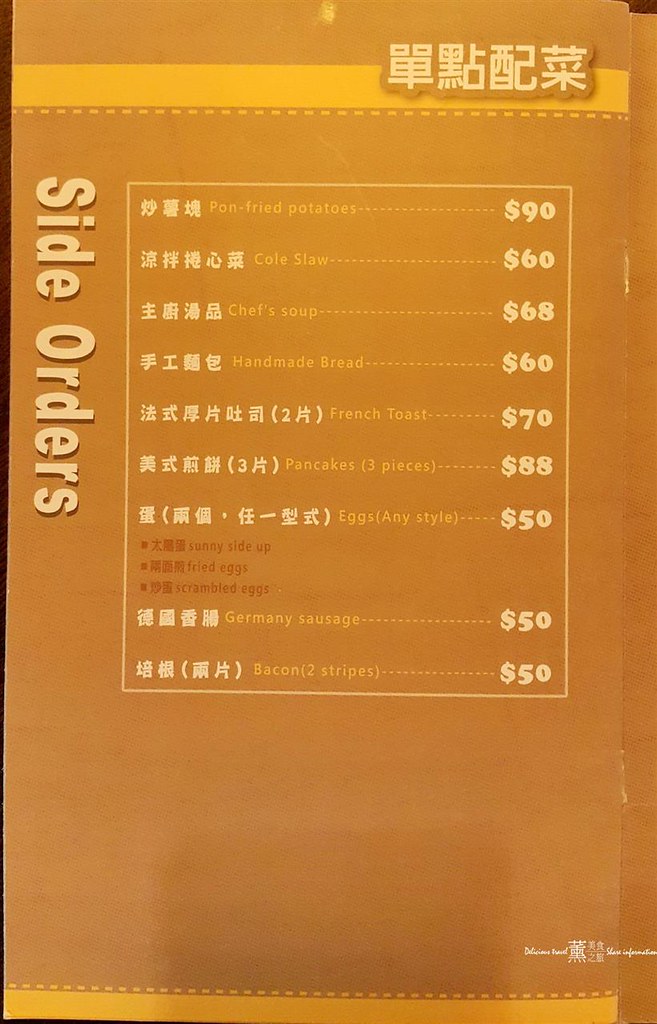A detailed and descriptive caption for the image could be:

"An elegantly printed menu on luxurious golden paper is held upright, showcasing various dishes available at the restaurant. The focus of the menu is an orange-yellowish box listing the items you can order, framed by side orders detailed on the left. In the top right corner of the menu, as well as beside each item in the box, are Chinese characters indicating the name of the dish. The central part of the menu presents a tempting array of offerings: pan-fried potatoes for $90, coleslaw for $60, chef’s soup for $68, handmade bread for $60, French toast for $70, pancakes (three pieces) for $88, and eggs (any style including sunny-side-up, fried, and scrambled) for $50, each with Chinese translations. The list continues with Germany sausage for $50 and bacon (two strips) for $50. The bottom right corner features white lettering with additional Chinese characters, possibly denoting the restaurant's name or trademark. Encasing the menu, both on the top and bottom edges, is a distinctive yellow bar about half an inch wide, bordered by dashed lines for an elegant touch."